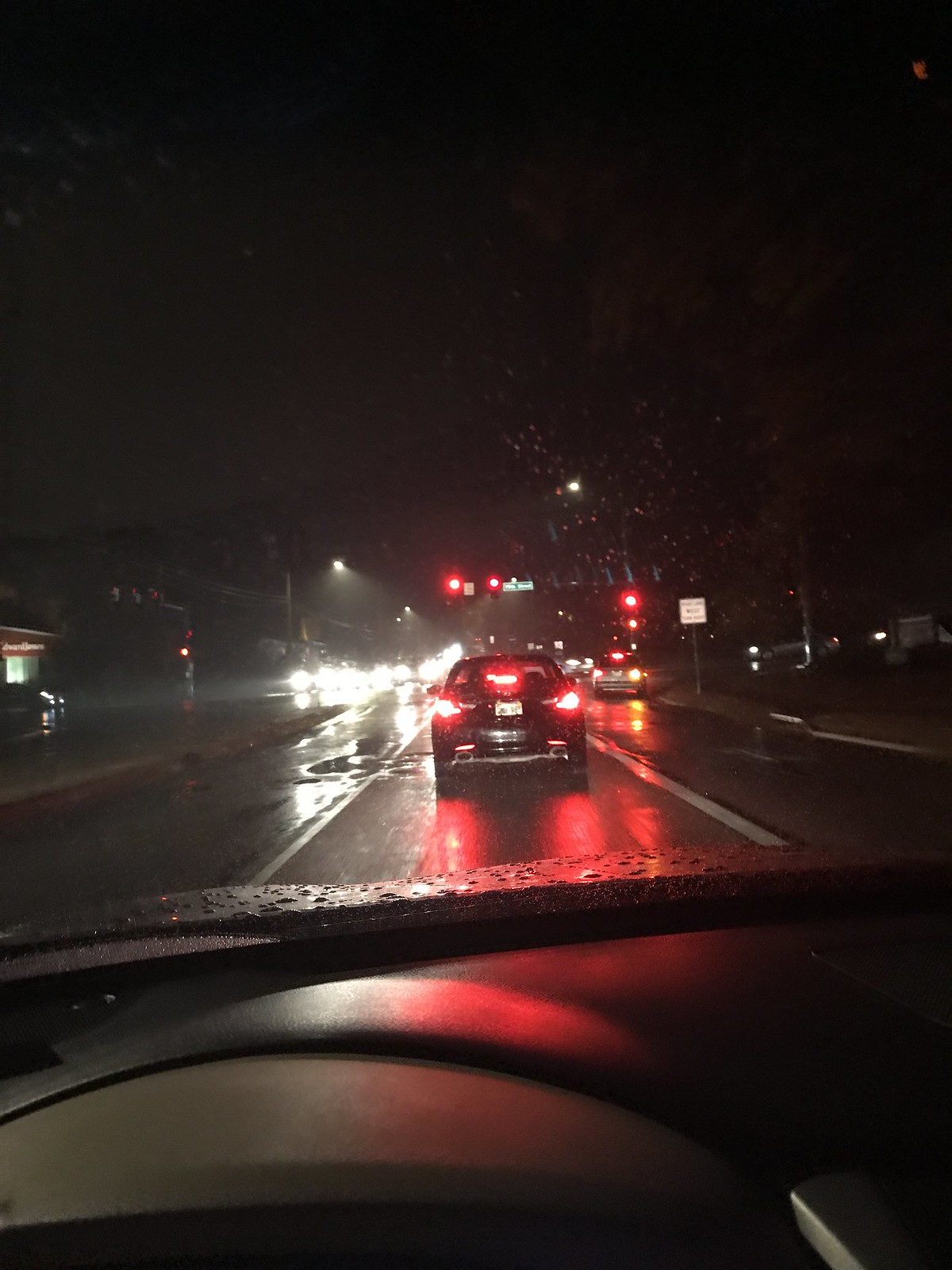The image captures a rainy nighttime scene from the perspective of a driver inside a vehicle, likely through a dash cam. The dashboard, covered in dark black plastic and featuring a windshield wiper streaked with raindrops, occupies the lower part of the image. Ahead, a black sedan with its brake lights on is stopped at a red traffic light. The slick, rain-soaked road reflects the illumination from street lamps and car headlights. On the right side of the road, there's a traffic light showing red, accompanied by a small green street sign that’s unreadable due to its size. The scene also reveals standing water on the pavement and several cars with headlights on, including one in the right lane possibly turning down a side street. Buildings flank both sides of the road, though they are indistinct against the dark, rain-streaked backdrop. The sky is pitch black, emphasizing the nighttime setting.